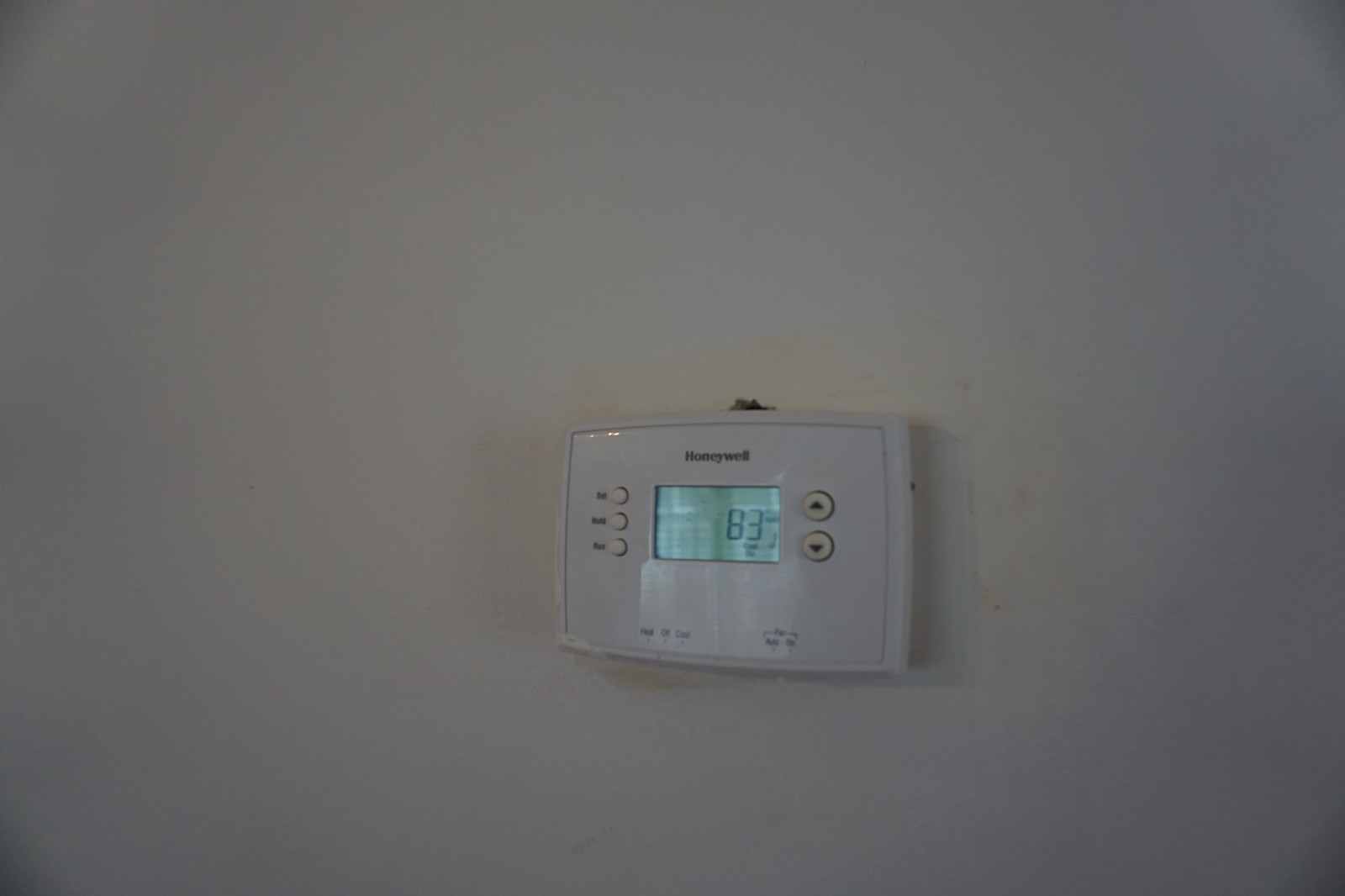A Honeywell thermostat is mounted on a white wall, slightly protruding with its shadow cast to the right. The device resembles a small box and features the Honeywell logo in black letters at its top. On its left side, there are three round, white buttons labeled "Set," "Hold," and an indistinct third label in black text. The bottom of the thermostat has three vertical black lines with three corresponding words and to the right of these lines are two additional words. Above this section is a rotated "L"-shaped line, extending up, then right, with a word in between, then continuing right and down.

The center of the thermostat has a bluish display screen showcasing the temperature, currently reading 83. To the right of the screen are two round, white buttons marked with black triangles facing up and down to adjust the temperature. At the top of the device is a black toggle switch for power control.